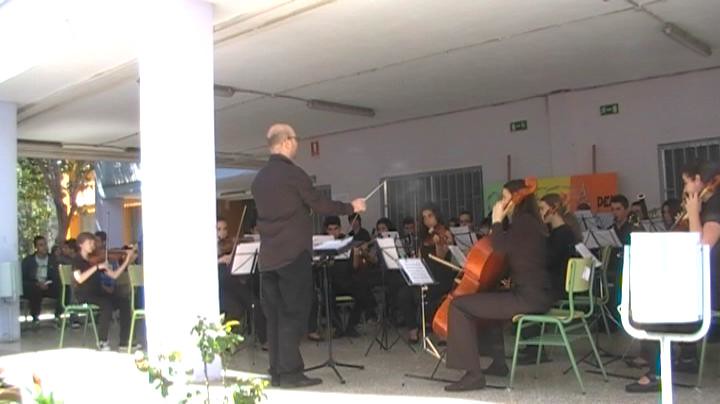The photograph depicts a school orchestra or band performing outdoors beneath a building's overhang or pavilion. The perspective is taken from behind the conductor, who is standing next to a white pillar on the left side of the image. The conductor, a white gentleman with a balding head and glasses, is dressed in a black button-up shirt, slacks, and black shoes. He holds a baton and stands by a podium with sheet music.

The orchestra members, appearing to be high school or college students, are all attired in black outfits and seated in green metal chairs. Each musician has a music stand with white sheets of music in front of them and their respective instruments, including a cello visible near the conductor. The area features a white roof and walls adorned with windows, suggesting they are performing in the courtyard of a school building.

The image includes some additional details, such as a few spectators in the distance and foliage visible at the bottom front. There is also a sign on a metal stand on the far right side, and various hanging objects from the ceiling that might be lighting or metal cylinders. The overall image is slightly low-resolution and blurry.